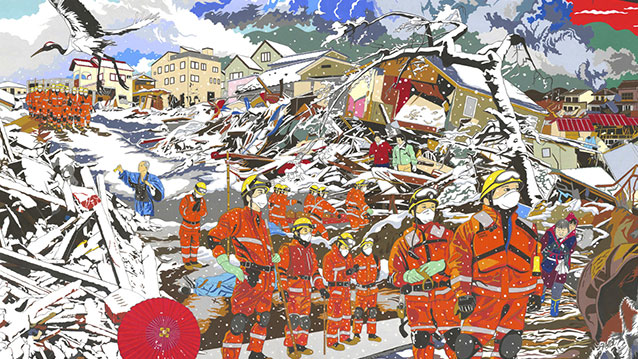The image depicts a vibrant, cartoon-style drawing of a chaotic scene in the aftermath of a snowstorm or earthquake. The foreground reveals extensive destruction, with shattered wooden structures and uprooted trees littering the landscape, while intact houses stand unscathed in the distance. Amidst the debris, numerous rescue workers, possibly firemen or emergency personnel, are diligently navigating the wreckage. These workers are dressed uniformly in reddish-orange suits, yellow helmets with resting goggles, and white face masks covering their mouths and noses. They are seen coordinating efforts as more workers approach from the background. A large crane bird soars across a cloudy, snow-filled sky, adding to the activity and urgency of the scene. Surrounding the chaos are neutral-colored buildings, tree branches, and distant mountains painted in blue, gray, and green hues, offering a contrasting calm to the disarray below.